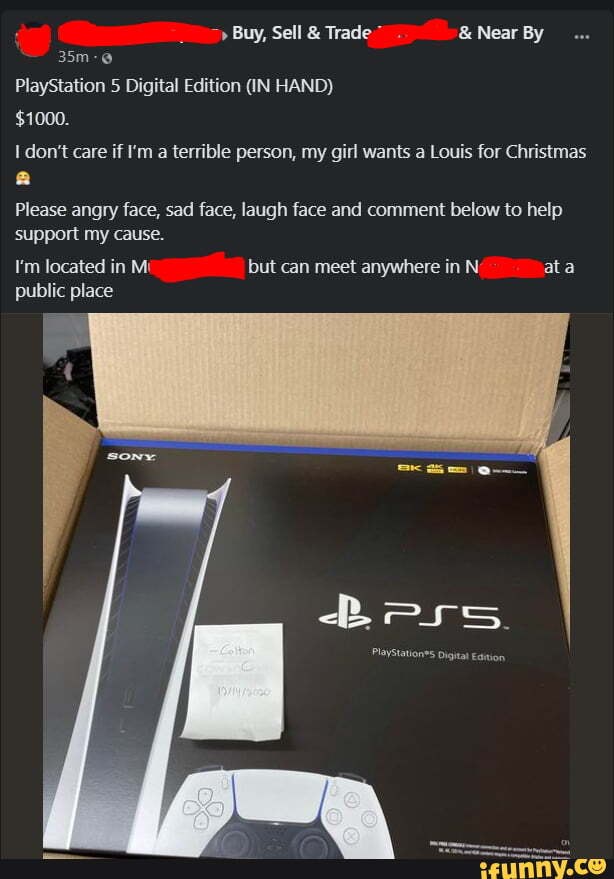**Caption:**

This image is a screenshot of a social media post with a black background. At the top, there is a profile picture obscured with a red marker, along with the name of the individual, also hidden with red ink. The post, made 35 minutes ago, advertises a PlayStation 5 Digital Edition available for $1000. The seller candidly admits, "I don't care if I'm a terrible person, my girl wants a Louis for Christmas," accompanied by various emojis depicting different emotional reactions. Additionally, the seller encourages viewers to comment to support their cause. The location details are redacted with red ink, but the seller mentions they are willing to meet at a public place. The post is punctuated with an image of the PS5 box. All the text in the image is written in white, while at the bottom of the screenshot, there is a watermark from ifunny.co in yellow text.